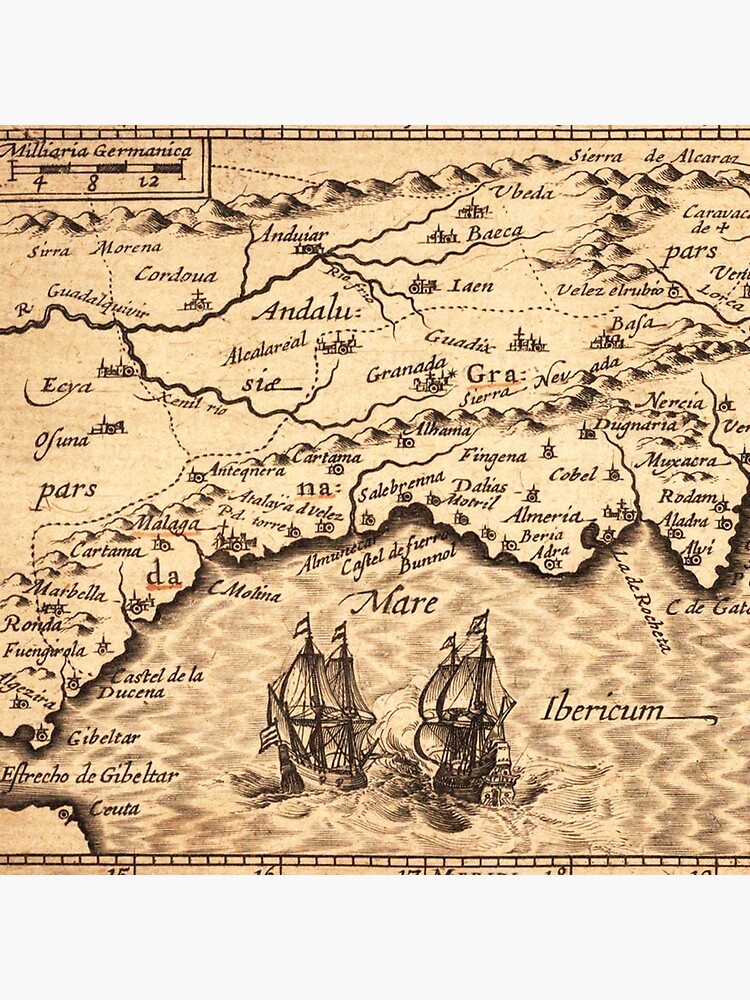The image is a square, old-style geographical map reminiscent of the Christopher Columbus era, framed with a thin white border at the top and bottom. In the top left-hand corner, the text "Militaria Germanica" is prominently displayed. The map showcases both land and sea, with the bottom portion depicting the ocean, shaded in a black Chevron style, where two large sailboats, sketched facing away from the viewer towards the shoreline, navigate the waters. In the sea section, the word "Ibericum" is inscribed. The land portion of the map is intricately detailed with solid and dotted lines indicating roads and mountain ranges. Numerous italicized place names such as Andalou, Granada, Baca, Fingenna, and Cordua, among others, are scattered across the map. The map also features a legend in the upper left corner, which includes scale indications at four, eight, and twelve units to represent distance.